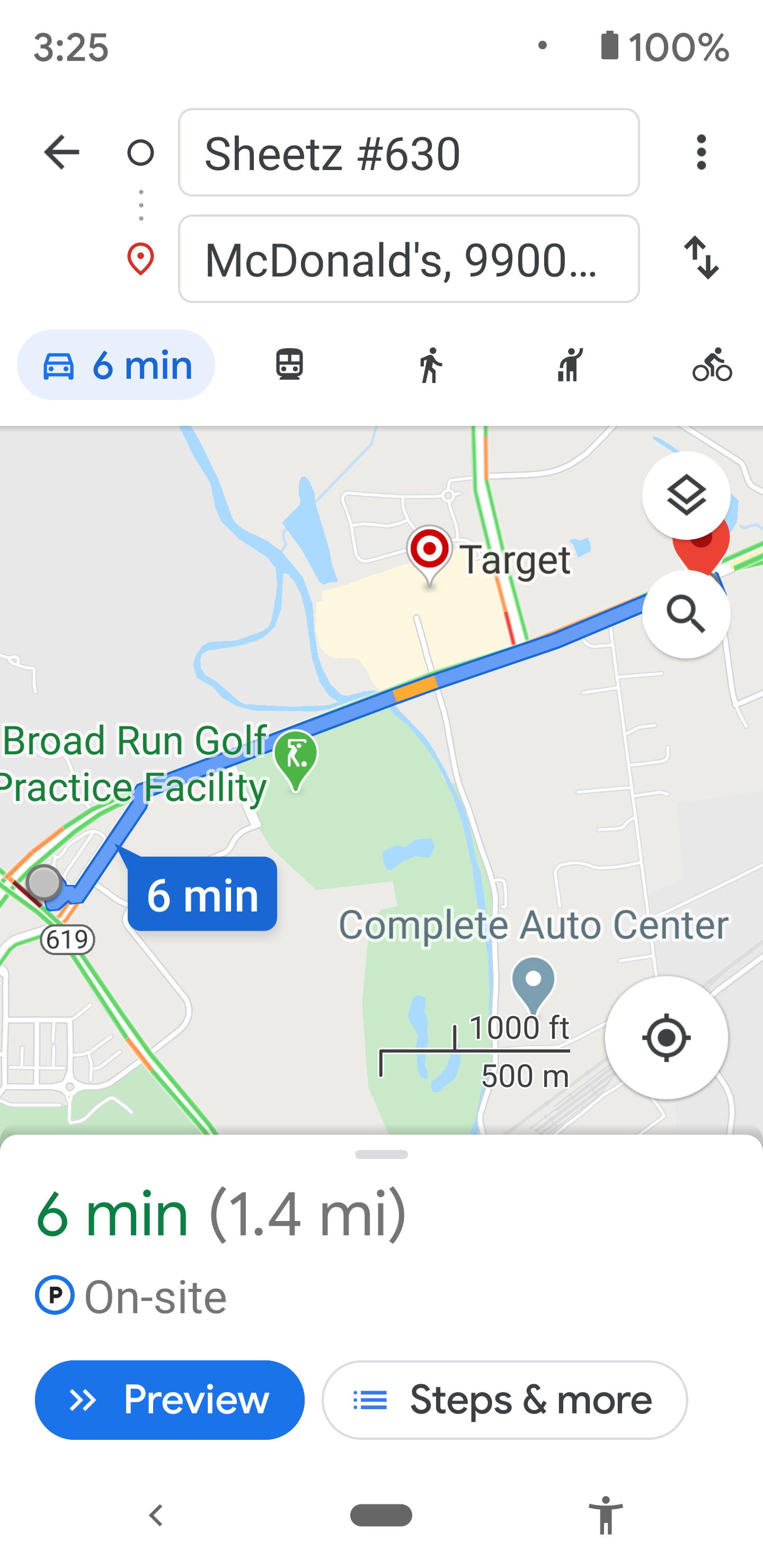The image depicts a screenshot taken on someone's smartphone while they were searching for a McDonald's location. At the top of the screenshot, the time reads 3:25 PM, and on the right side of this line, the battery icon indicates it is fully charged at 100%. 

An arrow pointing to the left and a circular icon labeled "sheets number 630" are also visible at the top. Just below, there's a red pin marking the location of McDonald's with the address truncated after "9900...". Beside the McDonald's pin, there's a car icon indicating it is a six-minute drive to the destination. Additionally, options for walking, biking, or taking the bus are available.

The map displayed in the screenshot has a beige background with green regions representing forests and other green areas. Points of interest, such as a Target store and the Broad Run Golf Practice Facility, are also marked on the map. The route to McDonald's is indicated, showing that the distance is 1.4 miles. Further details include on-site information and a preview, with a prompt for "steps plus more" to navigate the route.